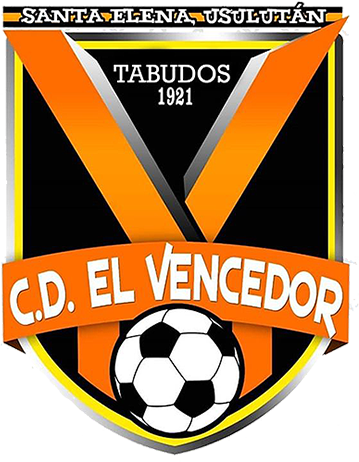The image features the logo of the soccer team CDL-Vencedor, prominently centered on a plain white background. The logo itself is designed in the shape of a shield with a rounded, pointed base. At the top, against black and orange horizontal stripes, the words "Santa Elena Usulutan" are displayed in white lettering. Below this, a large orange 'V' dominates the center of the shield, set against a black background and outlined in yellow. Beneath the ‘V’, the word "Tabudos" appears in white text, followed by the year "1921". An orange banner runs horizontally below this, inscribed with "CDL Vencedor" in white letters. At the bottom of the shield, there is a black and white soccer ball, completing the design. The color palette includes white, orange, black, and yellow, adding dynamic contrast and visual interest to the logo.